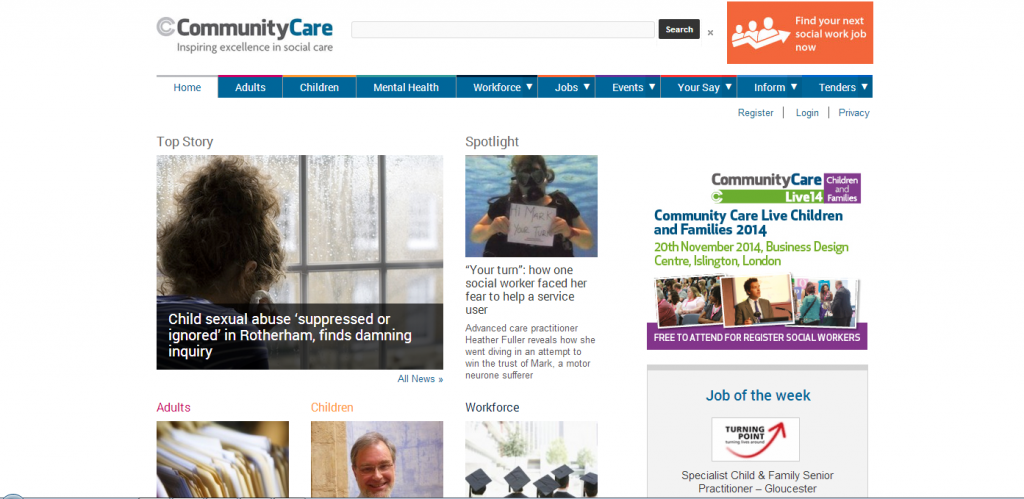Screenshot of the Community Care Website: 

The screenshot showcases the homepage of the Community Care website, whose tagline is "Inspiring Excellence in Social Care". At the top, there is a search bar where users can input their queries and click the search button, accompanied by an "X" icon for quick deletion of text. An eye-catching orange box with the prompt "Find your next social work job now" is prominently displayed. The website has various tabs such as Home, Adults, Children, Mental Health, Workforce (each with a dropdown menu for further options), Jobs (dropdown), Events (dropdown), Your Say (dropdown), Inform (dropdown), and Tenders (dropdown).

Beneath these main tabs, users can find options for Registering, Logging In, and reviewing Privacy settings. The site also features several highlighted stories aimed at engaging users. The top story is titled "Child sexual abuse suppressed or ignored in Rotherham, finds a damning inquiry." Another spotlight story shares a personal narrative: "Your Turn: How one social worker faced her fear to help a service user," detailing Advanced Care Practitioner Heather Fuller's underwater dive to earn the trust of Mark, a motor neuron sufferer.

Additional sections include Community Care updates, with features like "Job of the Week: Specialist Child and Family Senior Practitioner," and sections dedicated to Workforce, Children, and Adults.